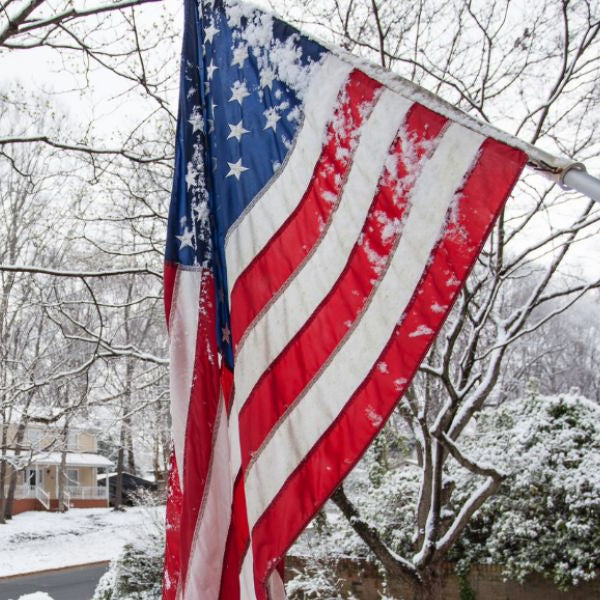This outdoor photograph captures a close-up of an American flag hanging downward from a silver flagpole that protrudes from the right side of the frame. The flag, adorned with stars and stripes of red, white, and blue, is lightly dusted with snow. Surrounding the flag is a winter landscape featuring leafless deciduous trees and snow-covered bushes as well as a snow-covered wall. In the background, a beige and white two-story house with a brown base and white railings stands across a plowed street, which contrasts with the snow-covered sidewalks leading up to the houses. The house has a black door and the overall scene suggests the stillness of a fresh snowfall beneath a white sky, with hints of blue indicating the early morning light.